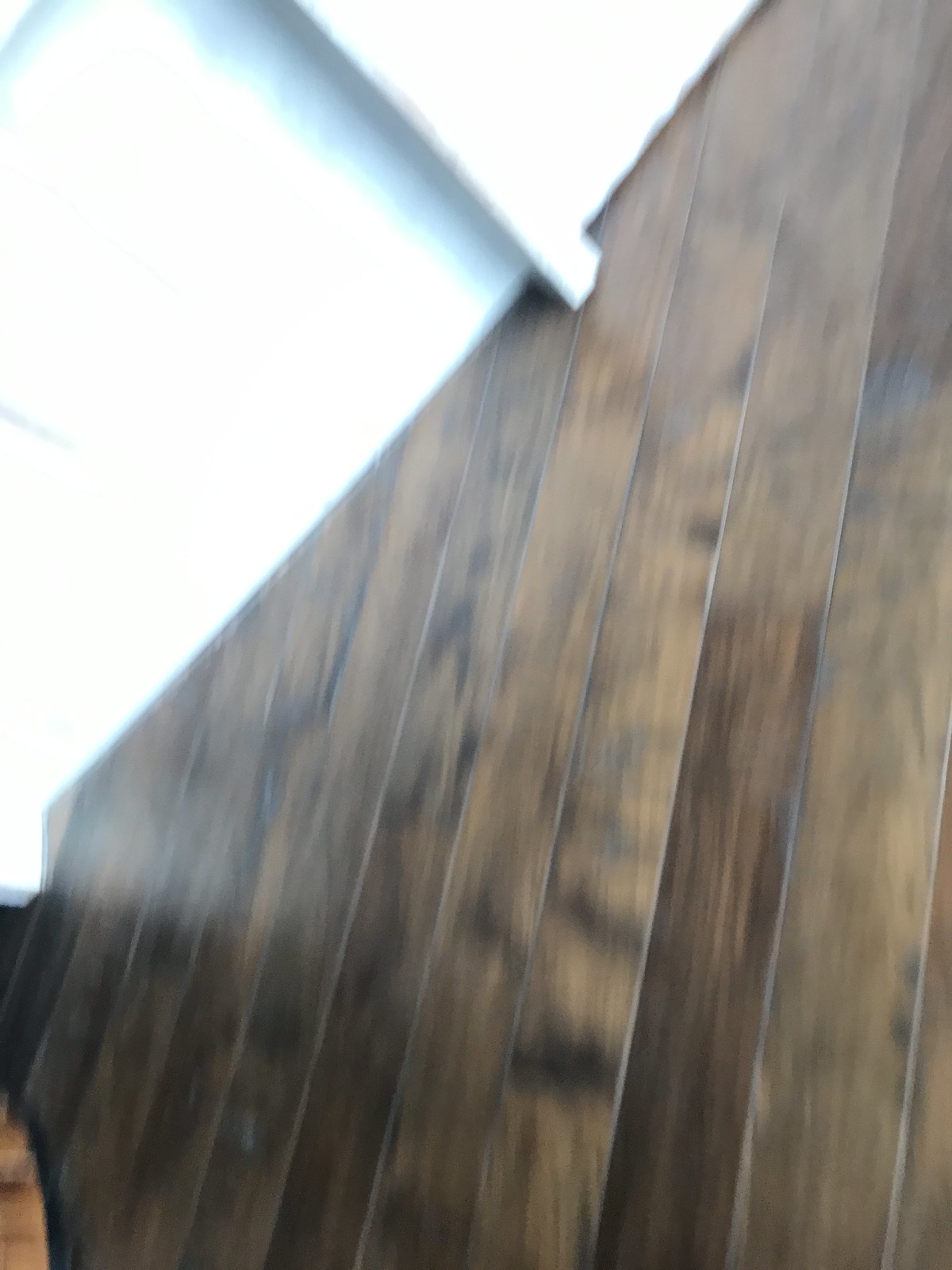This photograph depicts a section of an indoor space characterized by its distinct flooring and wall features. The floor consists of vertical wooden panels arranged in one-foot-wide strips, cutting at a diagonal angle where they meet the adjacent white wall. The paneling displays a rich wood grain that transitions fluidly from tan to medium brown to dark brown, creating a gradient effect. The blurred photograph shows some lateral bands of dark, possibly grayish-black hues splashed throughout the wood, indicative of the natural wood pattern.

The white wall behind the flooring is notably bright, possibly due to intense lighting that causes it to appear almost blown out in the image. There is a white support column visible about halfway up the photo, running from the floor and up towards the top left, contributing to the sense of structural complexity. Additionally, there seems to be what looks like a peeling white painted bracket or an element slightly detached from the wall, exposing a strip of blue underneath. This peeling element adds a layer of visual texture and intrigue.

Moreover, there is a mention of an angular beam cutting into the paneling lower on the wall, further enhancing the geometric interplay within the scene. A black-bordered object with a very tan surface is noticeable at the bottom left corner, its purpose or nature unclear, adding a sense of curiosity to the composition. Overall, the photograph captures a highly detailed and textured intersection of floor and wall, set at intriguing angles, under strong lighting conditions.